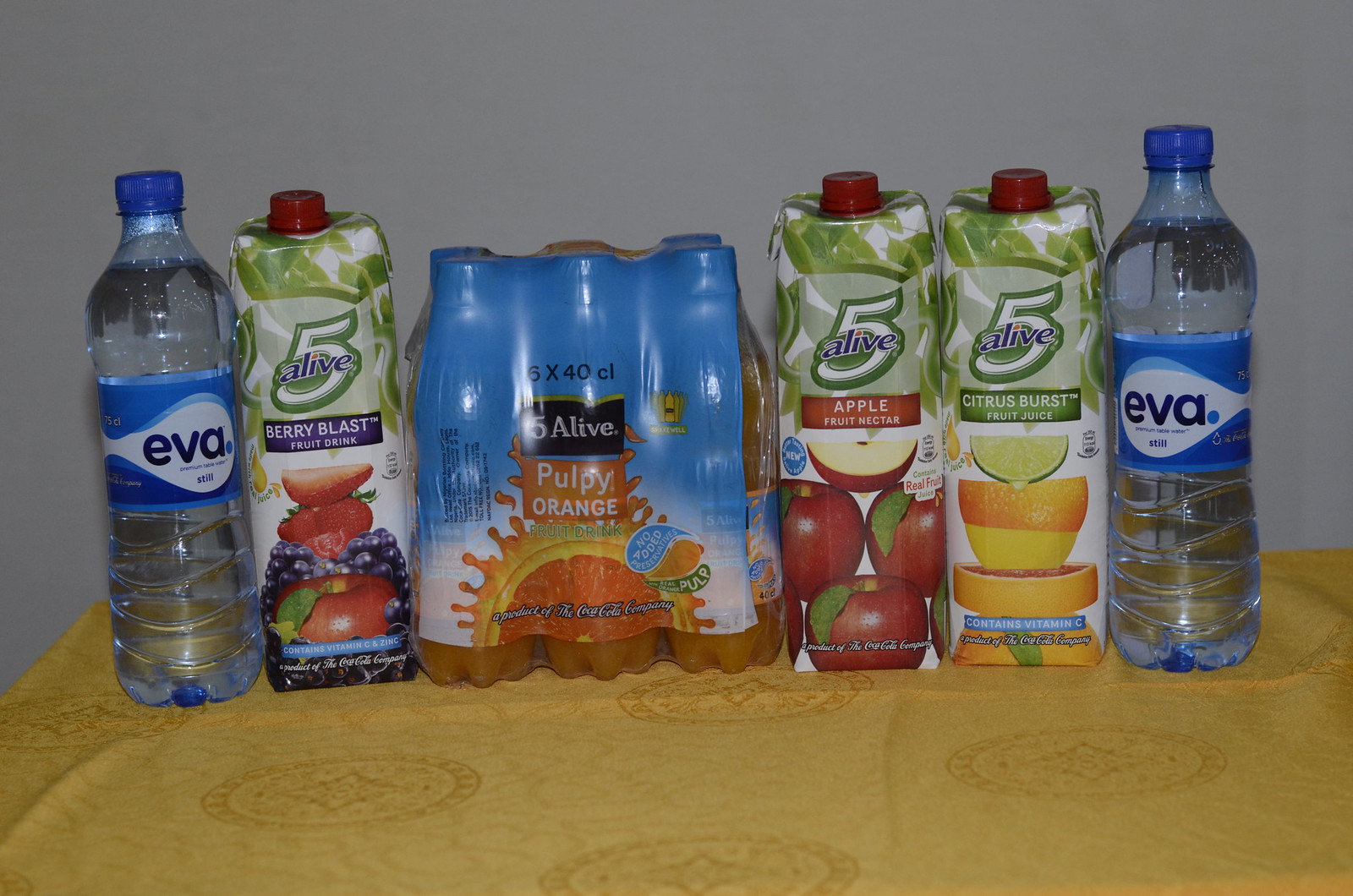The photograph showcases an arrangement of beverages on an indoor table covered with a gold tablecloth featuring circular patterns. Central to the display are various Five Alive drinks, including Berry Blast, Pulpy Orange (in a six-pack of bottles), Apple Fruit Nectar, and Citrus Burst. Each Five Alive drink prominently features the brand's logo and respective fruit illustrations on the packaging. Flanking the Five Alive drinks on either end are clear Eva water bottles, identifiable by their blue caps and distinctive EVA logo with a white droplet. The entire setup is against a light-colored wall, creating a balanced and visually appealing layout of vibrant and refreshing beverages.